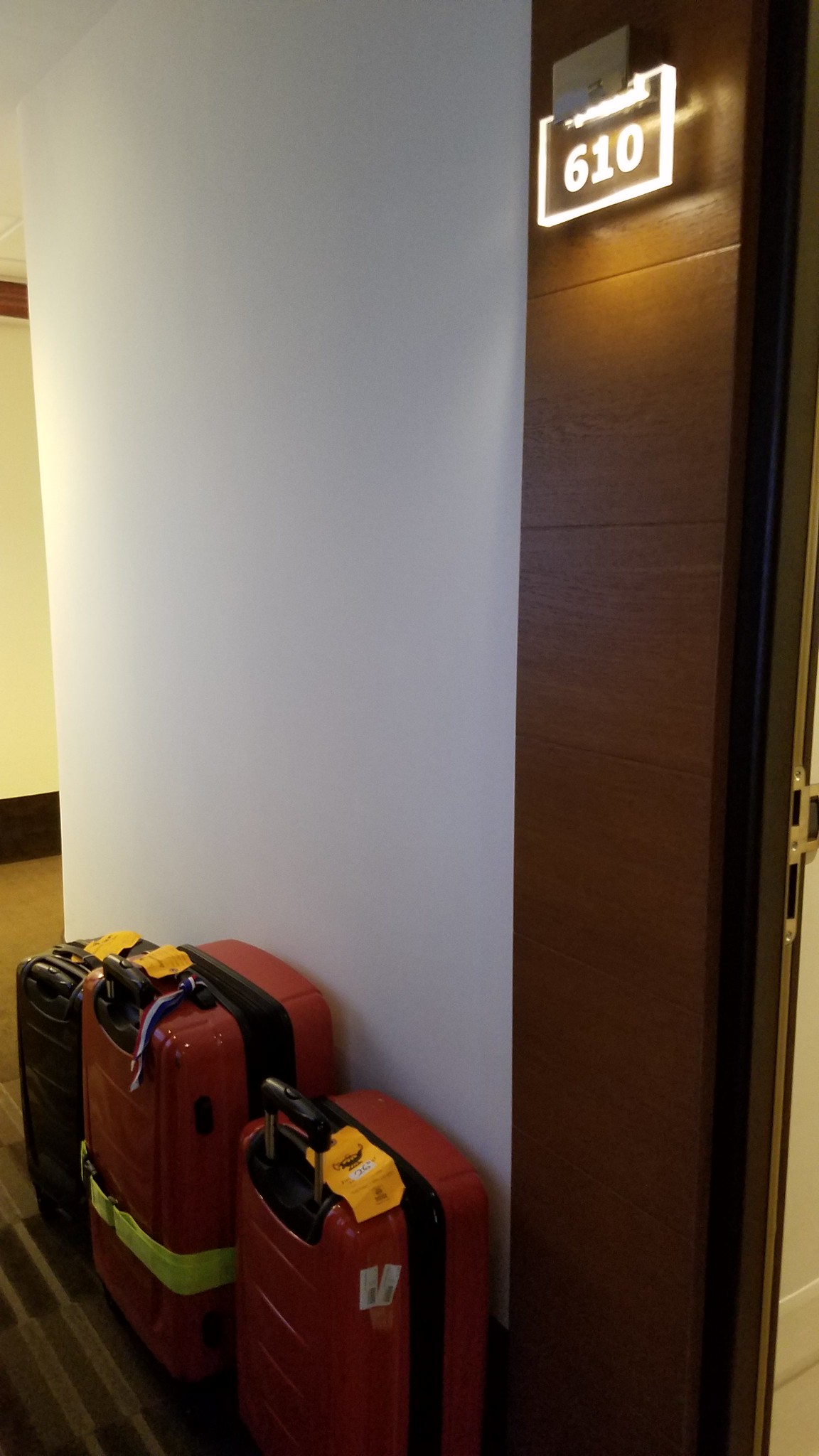This image captures a dimly lit motel hallway centered around a solid white wall and contrasted by a dark brown strip running vertically along the right edge of the picture, marking the boundary of a barely visible door off-frame. At the top of this brown strip is an illuminated acrylic sign displaying the room number "610" in white. The sign is subtly backlit, casting a soft glow on the number. Positioned at the bottom left of the frame against the white wall are three pieces of luggage, arranged side by side. The two red hard-sided suitcases stand prominently next to a smaller black one, all bearing evidence of recent travel with airline baggage check tags and yellow straps, and the closest bag displaying various stickers. The patterned carpet underlines the typical motel hallway setting, suggesting that guests are in the process of checking in or getting settled into their room.